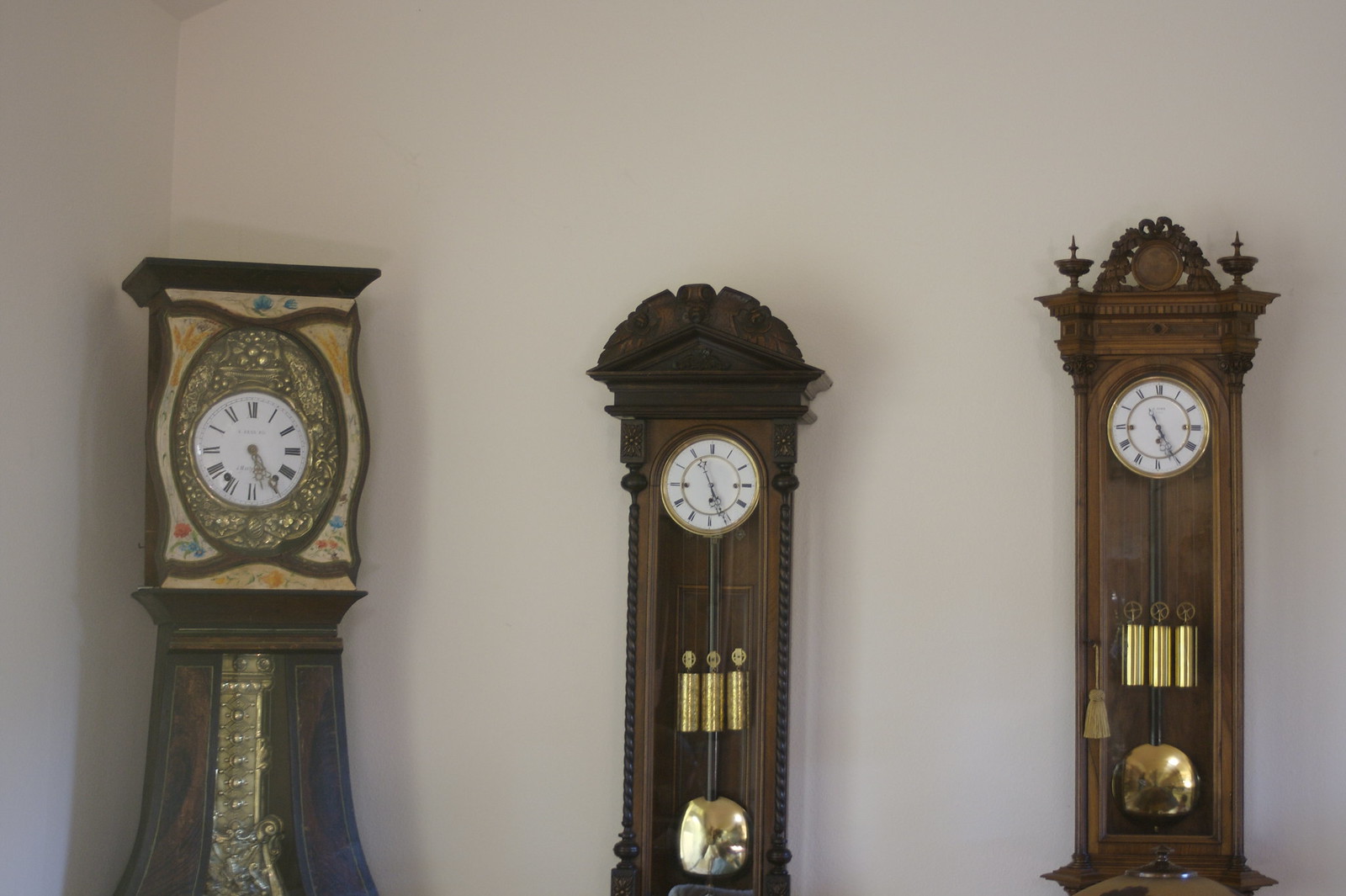The image displays three ornate antique clocks, positioned in front of a plain white wall indoors. Each clock features a blend of rich architectural details and functional design elements that highlight their historical significance and aesthetic appeal.

1. **Left Clock**: This clock is the most ornate of the three, featuring a thick and richly decorated structure. It has a gold-rimmed circular face adorned with black Roman numerals on a white background. The wood around it is a tan color with hints of floral patterns, though these details are slightly blurred due to distance. This clock also features an ornate gold section below the face, possibly framing a bell or pendulum.

2. **Middle Clock**: The middle clock has a taller, slimmer design with a rounded top leading into a long rectangular body. Its face is small and similarly styled with Roman numerals on a white background. The front panel is clear glass, revealing the pendulum and weights inside, all of which are gold-colored.

3. **Right Clock**: This clock, slightly lighter in wood shade, is also tall and slender but distinguished by more intricate decorative details, including turrets and floral carvings at the top that evoke a church-like appearance. Positioned in the corner, it features a round face within an ornate setting, and like the others, displays a gold-colored pendulum and weights.

All three clocks appear to indicate a time between 5:00 and 5:25, and cast subtle shadows on the wall behind them.